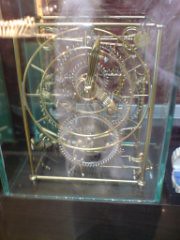The photograph depicts a small, intricately crafted mechanism encased within a clear glass or plexiglass cube, which stands on a reflective dark wood surface. The centerpiece is a meticulously detailed clockwork structure, primarily composed of gold and silver metal bars and gears. The gold-colored frame forms a skeletal outline, revealing the inner workings, including various cogs and a clock face adorned with gold hands. The see-through design allows for a full view of the complex gear system, suggesting an astronomical or artistic quality, though its exact function remains ambiguous. The image, although small and somewhat low in quality, hints at a museum display vibe with its elaborate craftsmanship and the prominent reflection on the glass case.